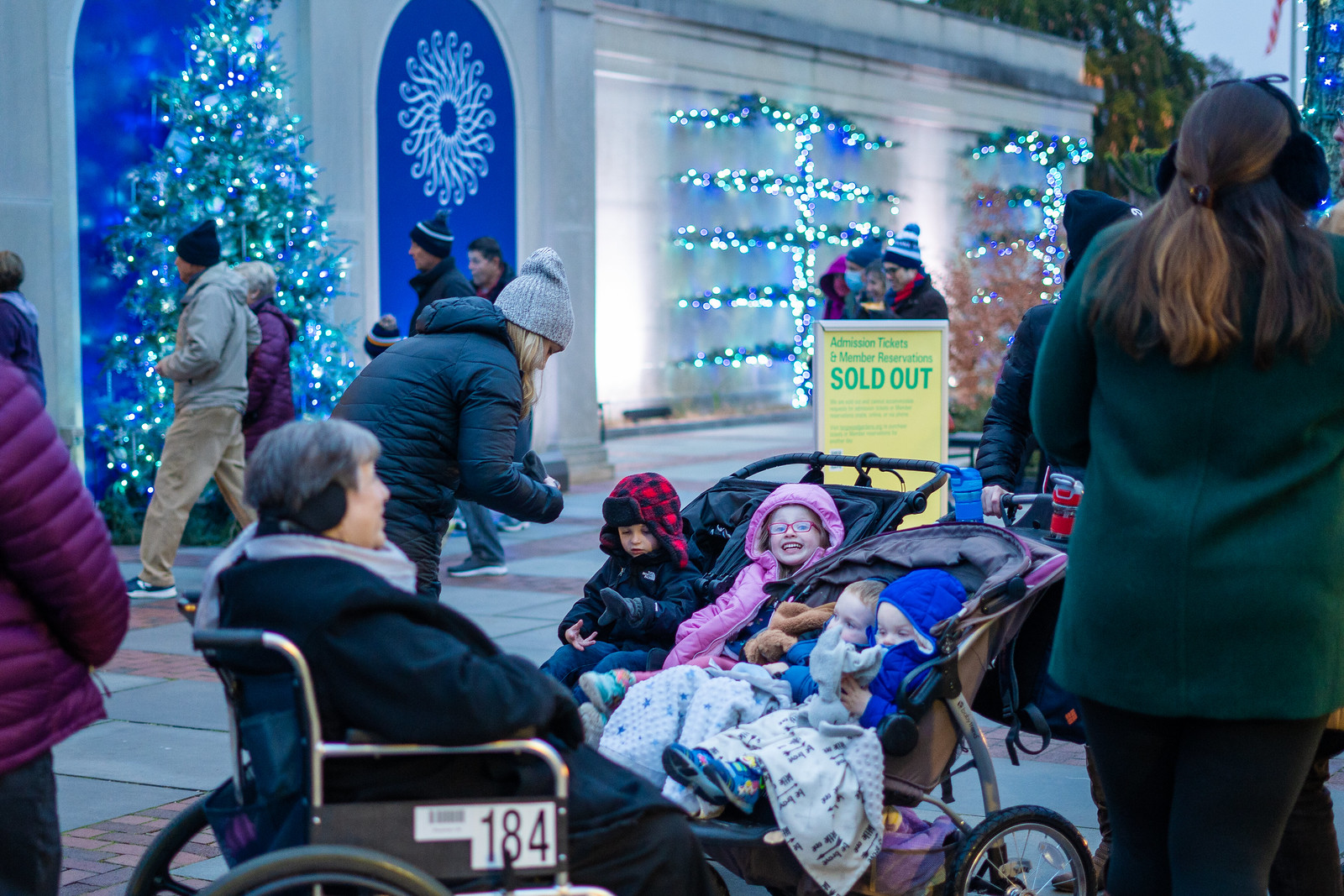The photograph depicts a bustling outdoor winter scene set around Christmas time, centered in front of a large white building festooned with blue holiday lights and green wreath decorations. The scene is lively, with many people milling about in warm clothing—jackets, earmuffs, hats—suggesting a cold day. On the left side of the image, an illuminated Christmas tree with blue lights stands prominently.

In the foreground, near the center of the frame, are two strollers. The first double stroller holds two children who appear to be around six years old: a little boy wearing a plaid red and black wool hat and a girl with red-framed glasses and a pink jacket. The second stroller contains two toddlers, likely around two years old, with one child partly covered by a blanket and the other in a blue jacket.

An older woman in a black jacket with black earmuffs is seated in a wheelchair positioned just left of center. She has gray hair and wears a weighty scarf, facing slightly to the right. The wheelchair features chrome handrails and a white label marked "184."

Behind the strollers, in the background, there's a notable yellow sign with green lettering that reads, "Admission tickets and member reservations sold out," indicating some kind of event. The scene is lively and captures the festive, bustling atmosphere of the holiday season with a mix of detailed decorations and warmly dressed individuals.